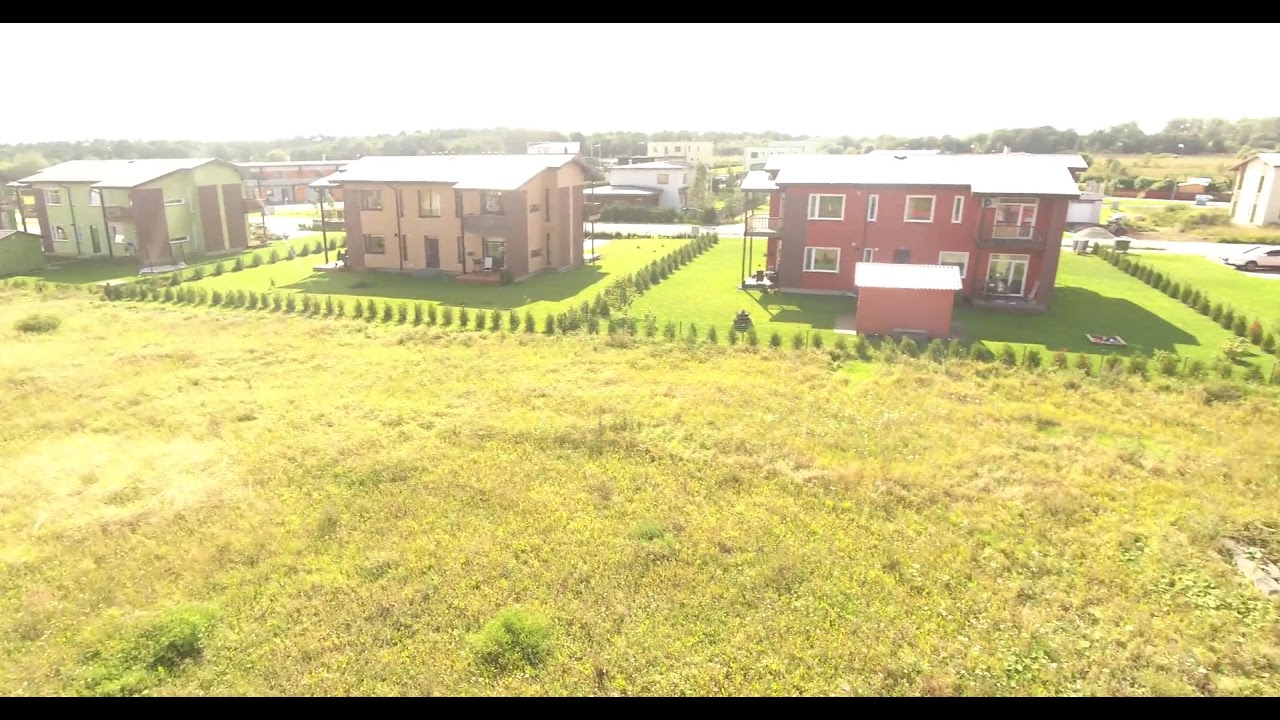The photograph, framed with a thin black header and footer, captures a slightly hazy and somewhat blurry view of a neighborhood, emphasizing a spacious, grassy area. In the foreground, there's a field of somewhat manicured green grass, not overgrown. Directly ahead, three distinct houses stand in a row: a red house with a shed, a beige house in the middle, and a white and brick house to the left. Each house is surrounded by neatly planted small ornamental evergreen trees that outline their square yards, conveying a sense of tidiness. The houses themselves appear to be about two stories high, with the roofs notably gleaming white. Beyond these homes, other residences and a road can be seen. The green grass, though lush, takes on a yellow-gold tinge, contributing to the picture's whitewashed, over-processed appearance. The entire scene unfolds under a gray sky, adding a muted backdrop to this tranquil neighborhood view.